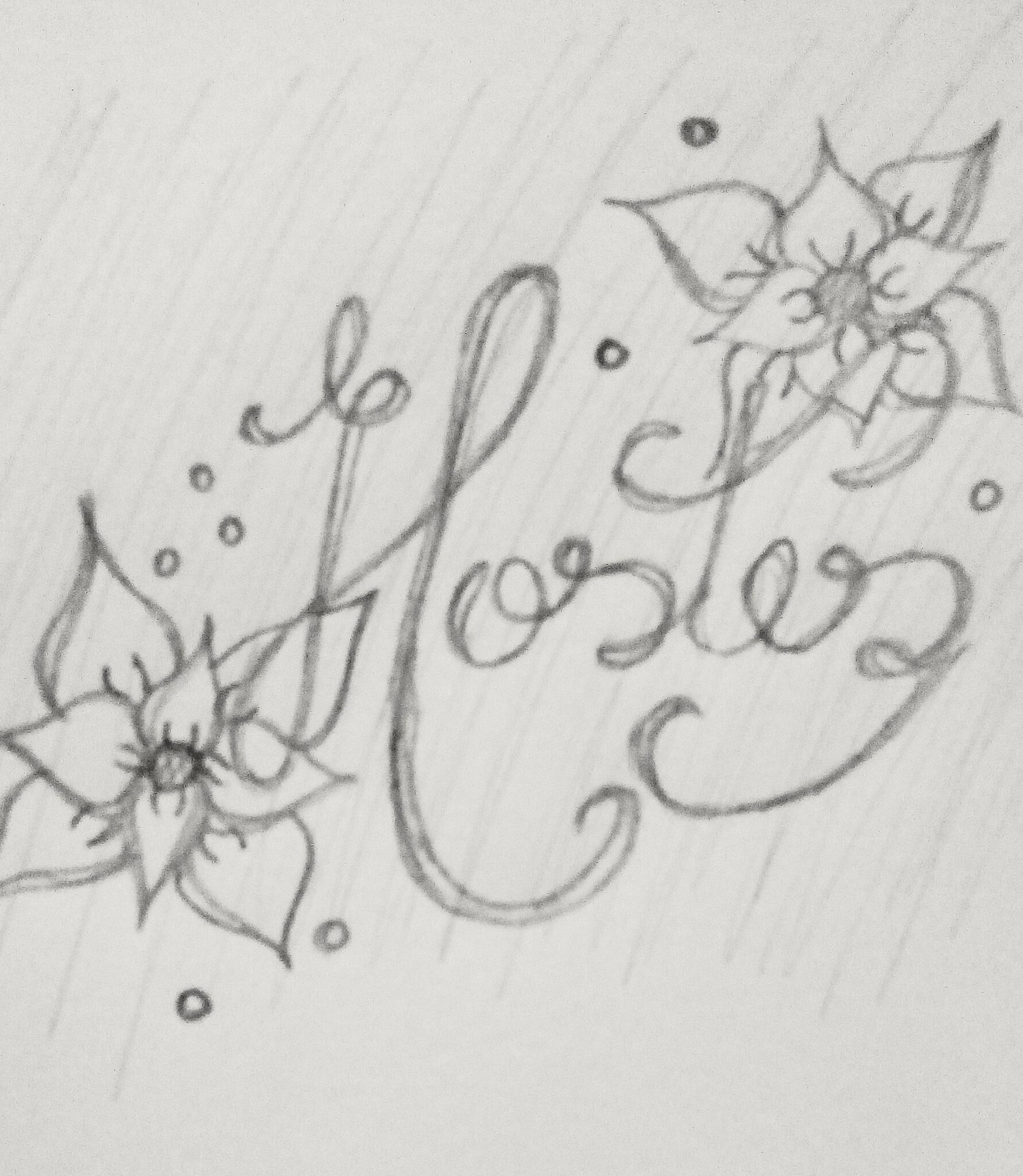The image features a white background with a meticulously detailed pencil drawing at the forefront. Dominating the composition are two flowers, positioned symmetrically to the left and right sides of the frame. 

The flower on the left displays a central circle surrounded by radiating lines, giving the appearance of a radiant sunflower or daisy. The petals extend outward in a dynamic, almost spiraling fashion, suggesting a sense of motion or growth. Similarly, the flower on the right mirrors this intricate design with identical features.

In the center of the image, a cursive signature provides an elegant touch, swirling gracefully across the space. The signature is somewhat illegible but appears to potentially spell "floss-tess" or a similar name, characterized by its elaborate loops and curves.

Additionally, the drawing is embellished with a series of pencil marks and small dots distributed around the flowers, adding a textured and intricate detail. Specifically, three dots are positioned above and two dots below the left flower, while the right flower is accompanied by one dot above, one to the side, and one at the bottom. These subtle elements enhance the overall texture and depth of the artwork.